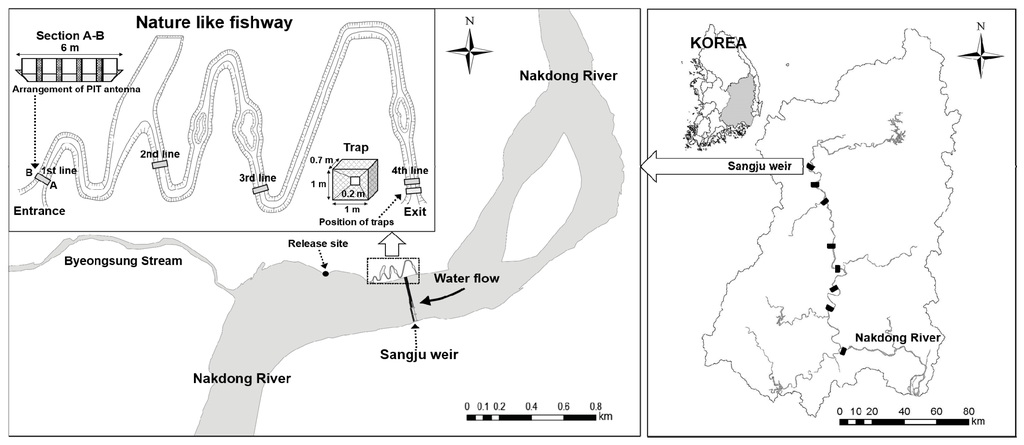This detailed map illustrates a nature-like fishway system embedded within the Nakdong River in South Korea. The map is divided into three smaller sections for clarity. 

The main section, located on the right, provides a comprehensive view of Korea, highlighting the Nakdong River which flows south through the country. This map includes a series of rectangles marking the locations of weirs, among which the Sangju Weir is specified, perhaps indicating dams or obstacles within the river. 

The second subset, indicated by an arrow pointing left from the label Sangju Weir, zooms into a segment of the Nakdong River characterized by two meandering bends. The river splits slightly before converging again, ultimately continuing its southward flow. In this section, the label “Nakdong River, water flow moving south” highlights the current's direction, and the 'Sangju Weir' is depicted bridging the river between these bends.

The third subsection offers a focused view of the nature-like fishway, adjacent to the Sangju Weir. This fishway is marked by a series of intricately arranged segments – labeled as the entrance, first line, second line, third line, trap, and fourth line – that facilitate the movement of fish. An arrangement of pit antennas is also shown, presumably employed to filter or control the fish movement, allowing them to bypass the weir and continue their journey along the river. The overall layout demonstrates meticulous planning to ensure aquatic life can navigate past artificial barriers seamlessly.

A north-south compass located in the top right corner, along with a legend depicting a scale ranging from 0 to 80 kilometers, aids in interpreting distances within the map. This detailed illustration provides insights into the geographical and artificial features of the Nakdong River, emphasizing the integrated nature-like fishway essential for preserving the natural aquatic ecosystem.